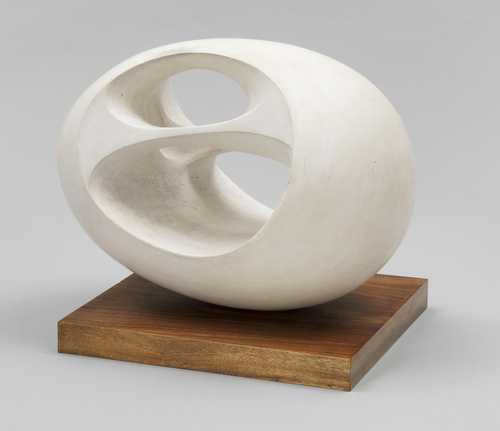This photograph features a white sculpture, likely made of ceramic, stone, or clay, which is shaped like an egg and artistically carved with several large, ovoid holes. The sculpture lies horizontally on a brown wooden stand, which is almost square in shape but slightly rectangular, matching the length of the sculpture. The egg-shaped piece has a smaller hole at the top and a larger oblong hole below it, with additional holes creating a sense of depth as they allow a view through the sculpture to the wall behind it. Positioned against a blank whitish-gray backdrop, the image captures the textured contrast between the smooth, hollowed-out sculpture and the wooden platform it rests on. The objects are displayed from a front point of view and appear prominently zoomed in, emphasizing their intricate details and the interplay of light and shadow.